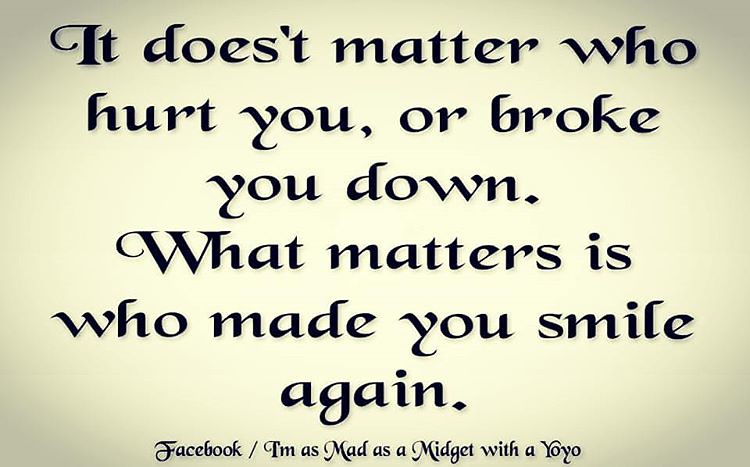The image is a rectangular text graphic with a background that transitions from light beige or yellow in the center to mid-gray in all four corners. The main text is printed in a slightly fancy, old black font, saying: "It doesn't matter who hurt you, or broke you down. What matters is who made you smile again." The formatting includes an error where "doesn't" is misspelled as "doe'sn't." Beneath this phrase, in smaller print, it reads: "Facebook / I am as mad as a midget with a yo-yo." The overall design is simple with the emphasis on the text, and the corners gradually darken, adding a subtle vignette effect.